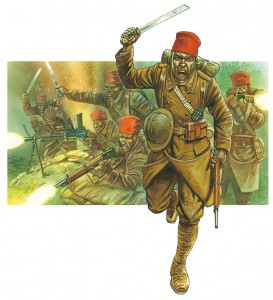The image is an illustration featuring a dynamic and vivid depiction of a soldier from the early 1900s, likely a member of the French mountain troops. The scene showcases a close-up of this soldier seemingly running out of the confines of a rectangular, historically-themed picture within the illustration. He is clad in a long green military coat and matching green pants, with boots that complete his uniform. His face is painted green, adding an intense, almost surreal element to his appearance. The soldier's right hand grips a machete raised high as if prepared to strike, while his left hand holds a rifle pointed downward. His red cap contrasts sharply with the green and brown color palette dominating the illustration, making it a focal point. Additional details include a grenade strapped to his chest and a helmet hanging from his waist. The soldier's expression is fierce, with his mouth wide open in a scream as he charges forward.

In the background, there is a rectangular image depicting a scene of battle, where numerous similarly dressed soldiers are positioned on a hill or behind a barrier. Some are firing rifles, with visible bursts of flame, while others raise machetes in the air, engaged in the heat of combat. The entire background scene maintains a loose color scheme of beiges, greens, and browns, creating a cohesive yet dramatic contrast with the white background that the central soldier breaks into. This artistic choice emphasizes the soldier's motion as he appears to leap from the historical frame into the viewer's space, encapsulating the chaos and urgency of battle.